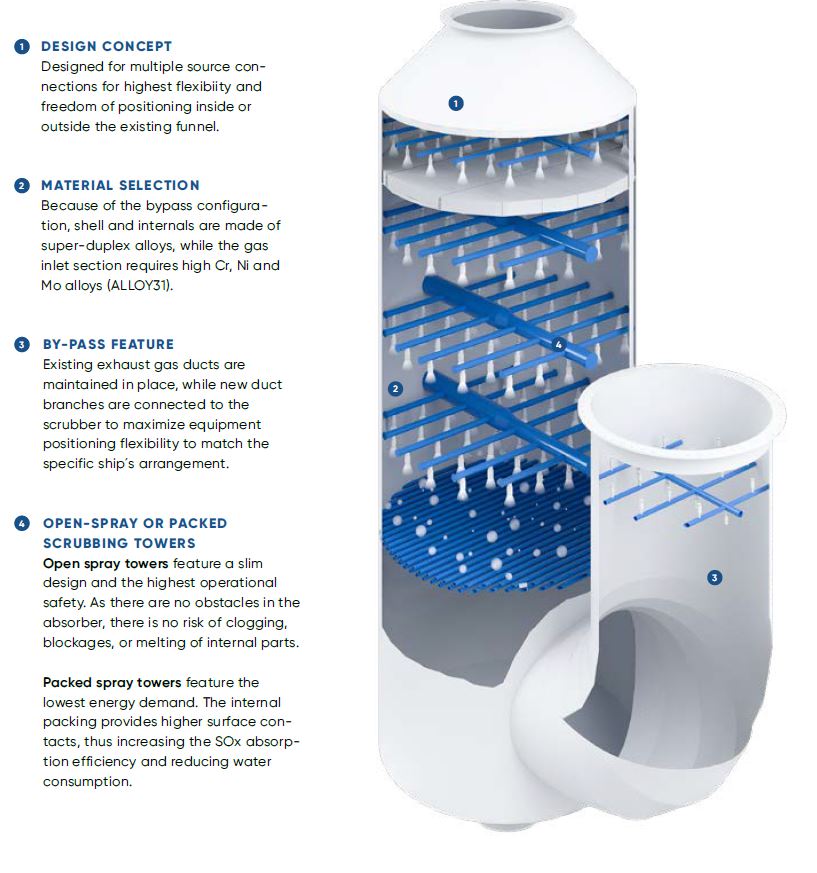This image features a detailed, cutaway view of a cylindrical filter system, showcasing its internal components and functionality. The central element is a vertically oriented main tunnel, depicted through a cutaway view that reveals crisscrossing blue strips and an intricate internal structure. This main structure is positioned prominently in the center, running from the top to the bottom of the image. To the bottom right, there's a smaller tunnel, accompanied by descriptive text.

The background highlights four key bullet points aligned on the left side, each delineated with blue numbering inside white circles followed by explanatory text:
1. **Design Concept:** This section describes how the filter is designed for multiple source connections to offer the highest flexibility and freedom in positioning, both inside and outside existing funnel systems.
2. **Material Selection:** It emphasizes the use of super duplex alloys for the shell and internals. The gas inlet section, requiring high CR, NI, and MO alloys, underscores the meticulous material choice to withstand harsh operating conditions.
3. **Bypass Feature:** This area provides a detailed explanation of the filter's bypass configuration that enhances its operational efficiency.
4. **Open Spray or Packed Scrubbing Towers:** It describes the design options available, including open spray towers and packed scrubbing towers, illustrating the versatility in application.

The design uses a color palette dominated by white, blue, and gray, giving it a technical, clean aesthetic. The image and accompanying text serve both as an instructional breakdown of the filter's design and a visualization of its internal mechanics, offering a comprehensive inside look at its operational framework.